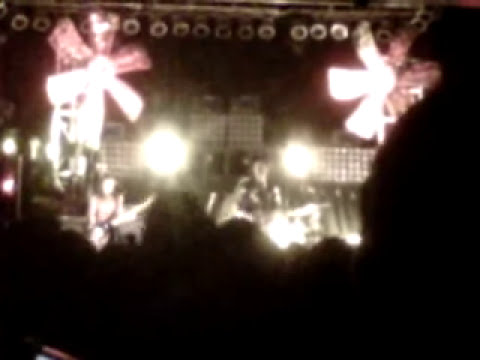The image captures a blurry, pixelated scene of a concert, taken from within the crowd. Dominating the foreground are dark silhouettes of concertgoers, backlit and indistinct, creating an anonymous sea of black blobs. The stage, set in pale yellow, black, and hints of light red and brown tones, features two guitarists: a woman on the left and a man on the right, illuminated by bright overhead lights. Flanking the stage in the top left and right corners are two large floral-shaped lights, each resembling a six-petaled daisy. Additional circular lights dot the ceiling, adding to the ambiance. The overall image lacks fine detail and textual elements, leaving an impressionistic view of the energetic concert atmosphere.